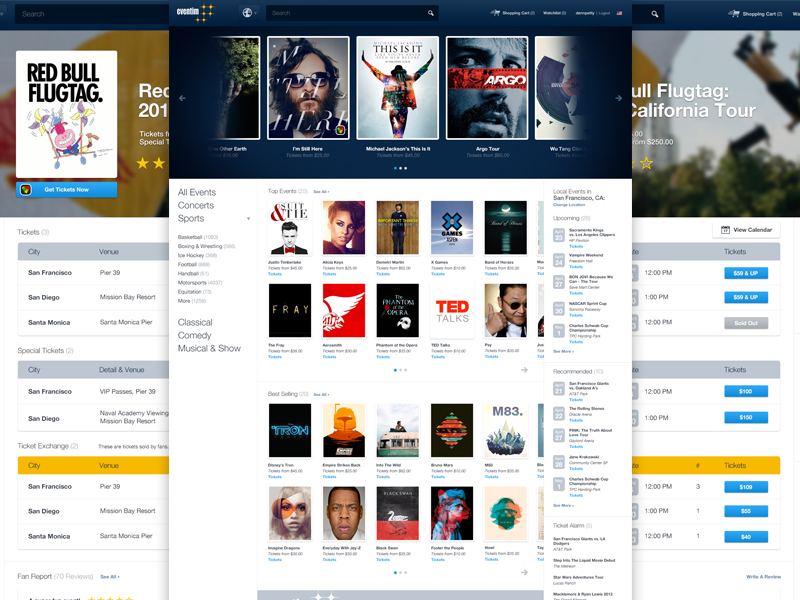The webpage appears to be a platform dedicated to both music and movies, featuring a diverse range of artists and titles. Dominating the top of the page is a reference to the Red Bull FLUGTAG event. Noteworthy mentions visible on the site include Michael Jackson’s “I'm Still Here,” the Argo Tour, Justin Timberlake, Alicia Keys, and the iconic musical "Phantom of the Opera." Additionally, there are references to Disney's "Tron," Imagine Dragons, the classic "Empire Strikes Back" from the Star Wars saga, and Bruno Mars. The text is exceptionally small, making it difficult to discern all the details and specifics. However, the general impression is that this site offers access to various music tracks and films, possibly highlighting top trending selections for users to explore and enjoy.